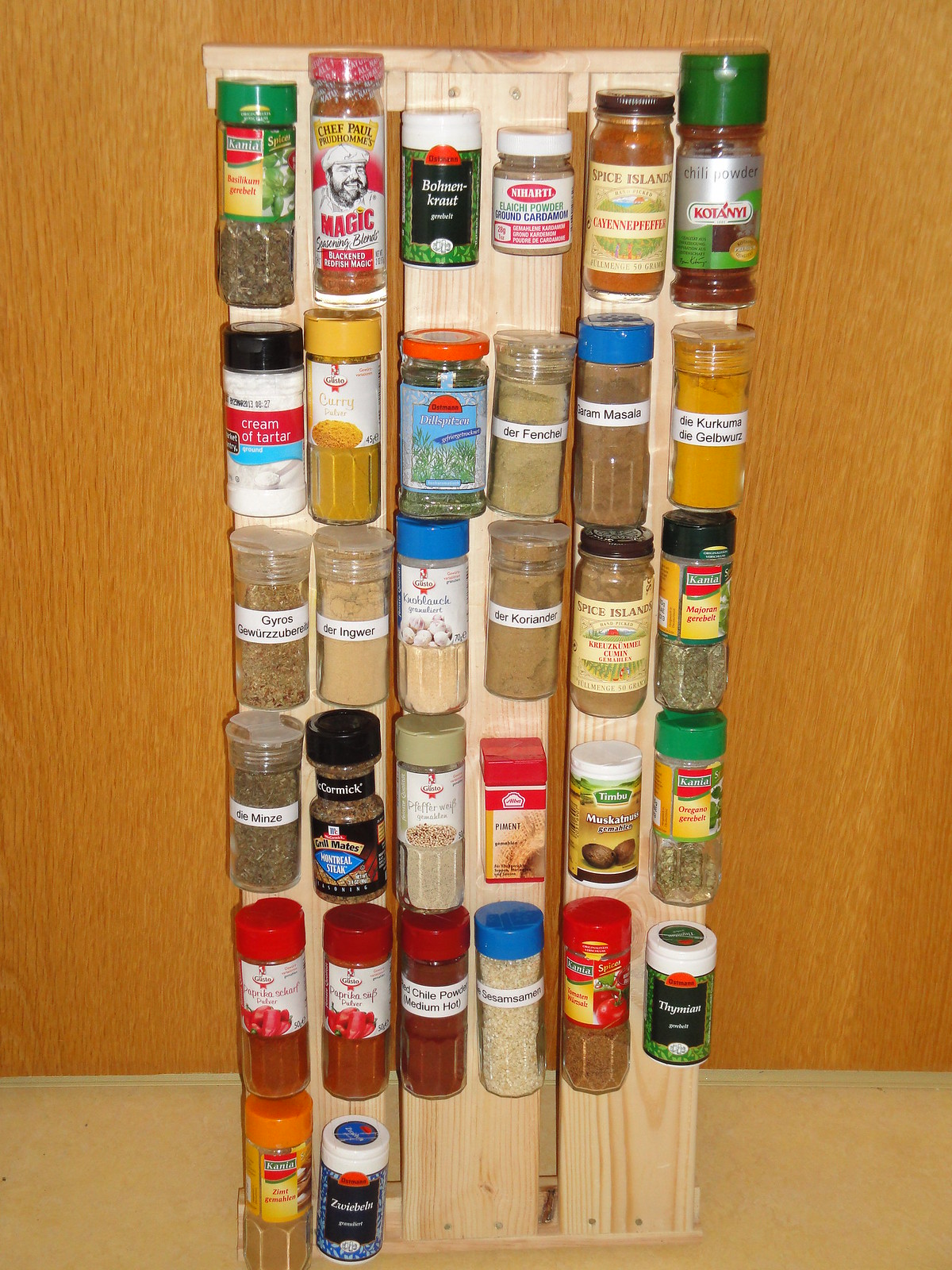The photograph showcases a meticulously crafted wooden spice rack, prominently placed on a light brown countertop and leaning against a light-paneled wooden wall. The rack is constructed from three vertical wooden planks, firmly nailed together, creating a visually appealing and functional display. These planks host an impressive variety of spices, housed in an array of containers that include glass jars, plastic bottles, and small tins. Notably, the spices include cayenne pepper, masala, gyro, garlic, thyme, cream of tartar, grilling spices, paprika, and various forms of onion. The containers are meticulously labeled, ensuring each spice is easy to locate. The spice bottles are arranged across five rows, with a sixth row featuring a couple of additional bottles, which appear to be effortlessly suspended as if floating on the rack. This organized and accessible collection of spices exemplifies practical homey charm against the rustic backdrop of the wood-paneled wall.